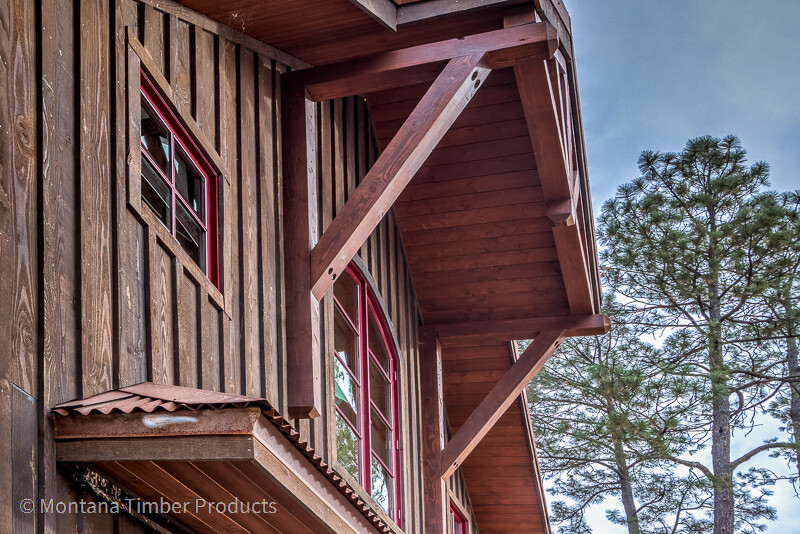The image captures the side view of a two-story wooden house, photographed from a low angle focusing primarily on the second floor. The house features dark brown wood siding, with the upper sections near the roof displaying more of a reddish-brown, cherry wood hue. Three distinct windows adorn the house: a square window on the left, a larger rectangular window near the bottom center, and another window at the very bottom which is partially cropped out. The windowsills are painted in a cherry red color. To the right of the house, two or three towering trees with green pine needles rise vertically against a backdrop of a blue to gray sky. In the bottom left corner of the image, small off-white text reads © Montana Timber Products. Additionally, an overhang supported by wooden posts, possibly 8x8 or 4x4, can be seen, which extends over what appears to be a covered porch area with a corrugated metal roof that shows signs of rust.